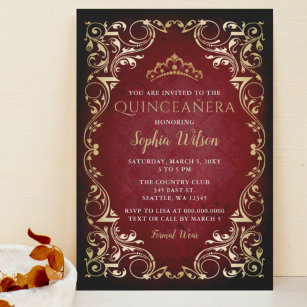This color photograph, taken in a slightly out-of-focus square format, captures an intricately designed invitation leaning against a wall. The invitation is for a Quinceañera honoring Sophia Wilson, held on Saturday, March 5th, from 3 to 5 PM at the Country Club, 345 East Street, Seattle, Washington. The invite features a glittery black background with ornate gold scrollwork along the borders, accented by jewel-like circles near the top and sides. Central to the design is a gold crown atop a dark red backdrop with the text "You are invited to the Quinceañera honoring Sophia Wilson" in elegant script. Additional event details are provided in white script text. An RSVP request is noted, asking to text or call Lisa by a specified deadline. The photo also includes a decorative white bowl filled with dried leaves in the bottom left corner, contributing to the overall aesthetic of the composition.